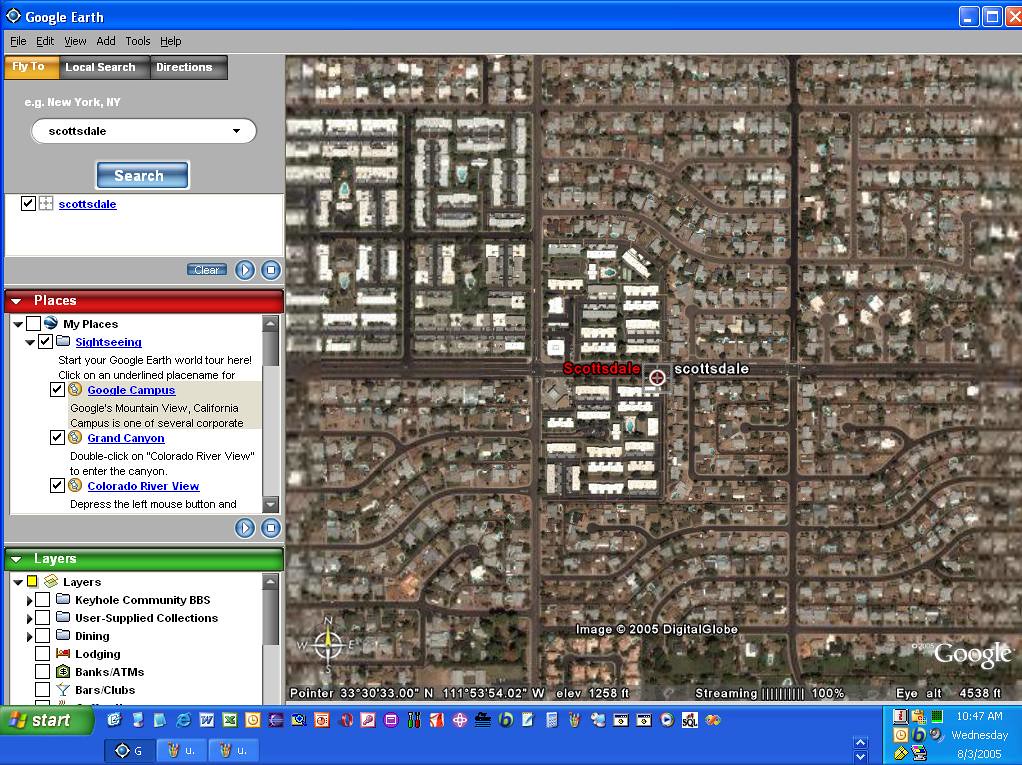This photograph captures a computer screen displaying a Google Earth map. The map appears to depict an area named Scottsdale, though it's uncertain whether this refers to Scottsdale, Arizona, or a specific street named Scottsdale. The map is divided into six sections, with buildings in some sections depicted in white, while others are colored in their natural gray-brown hues. 

On the left side of the screen, a menu is visible. At the top, it features options like "Google Earth," "local search," and "directions." The white search box at the top displays the text "New York, New York," with "Scottsdale search" written underneath. Further down, the menu lists categories such as "places," "sightseeing," "Google campus," "Grand Canyon," and "Colorado Riverview." Below these categories, there is another menu for "layers."

At the bottom of this sidebar menu, additional computer screen options are presented. In the bottom right corner of the screen, the word "Google" is prominently displayed in white letters.